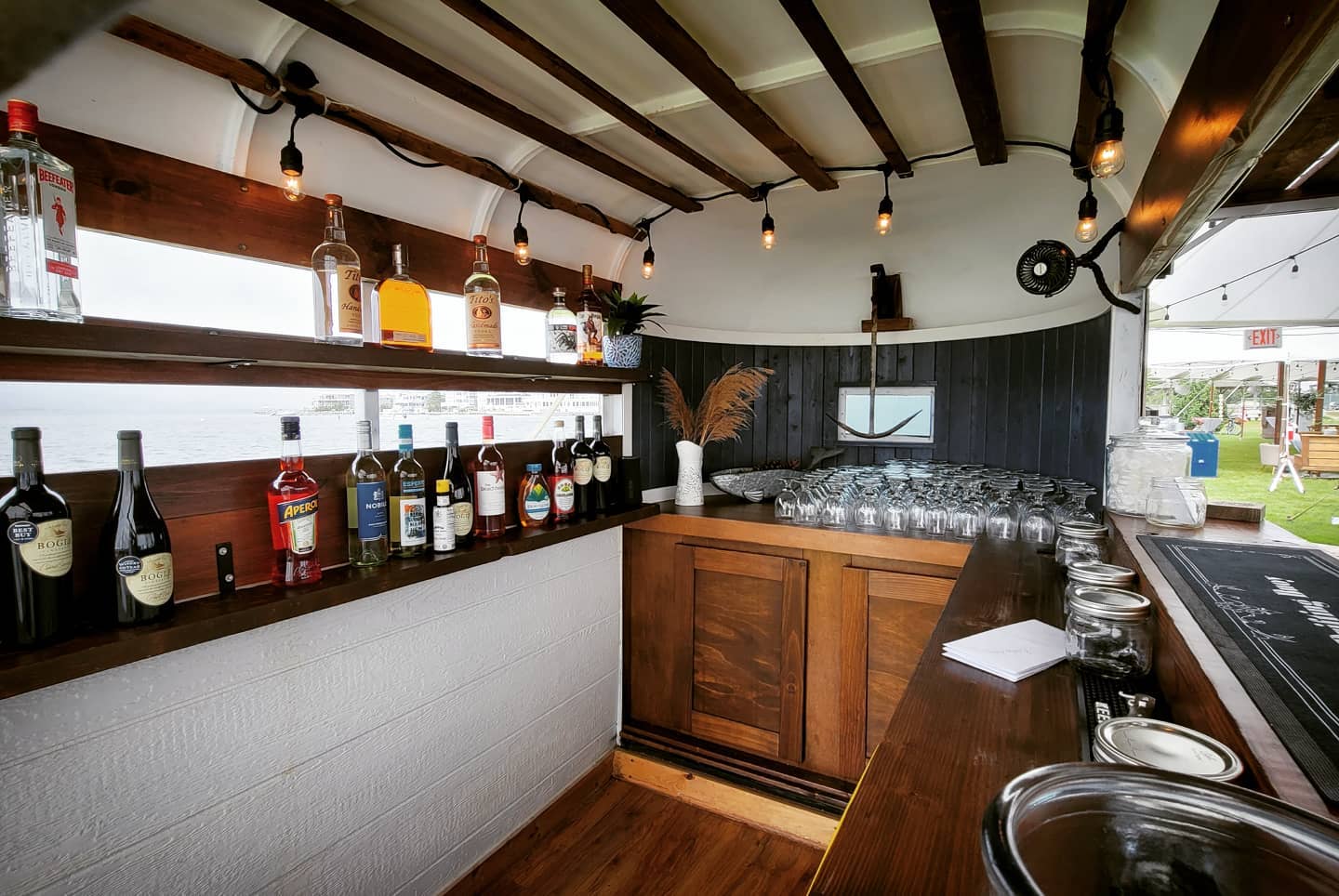This horizontal, rectangular image captures the interior of a bar with a slight distortion due to the camera lens, giving the room an unusual, stretched appearance. The back wall features shelves lined with a variety of liquor bottles, interspersed with notable gaps, suggesting a minimalistic or understocked bar. Below the shelves, an array of presumably clean glasses are neatly arranged, ready for use. The bar counter extends from the background toward the viewer, inviting patrons to approach. Through an open door in the back of the room, a vista of lush green grass is visible, potentially hinting at an outdoor event such as a wedding reception or a sports field where attendees might gather for refreshments during intermissions. The serene greenery and possible table setups outside contrast with the structured, indoor bar area, creating a versatile venue for social gatherings.